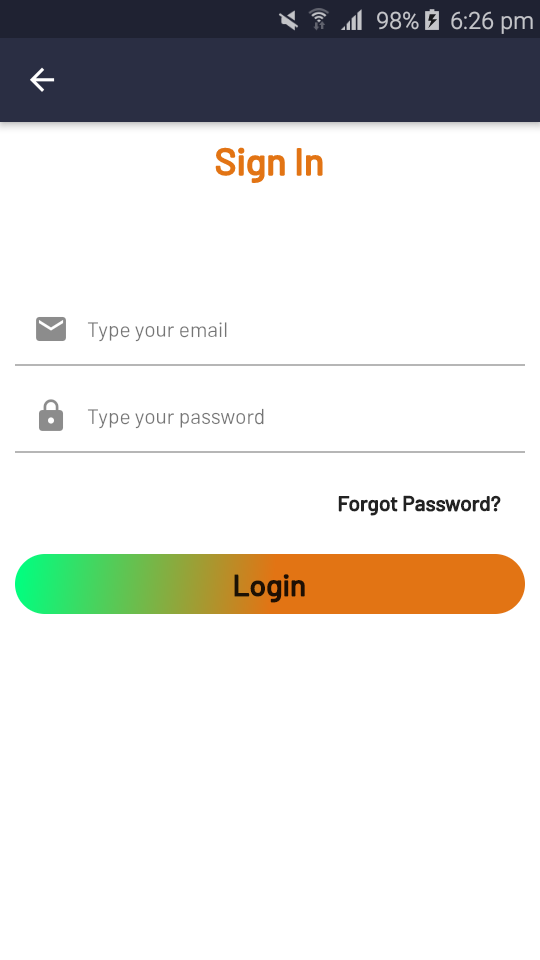In this image, we see a smartphone screen displaying the sign-in interface of a certain application. At the top of the screen, various status icons are visible: the time is 6:26 p.m., the battery is at 98% and charging, the network signal is full bars, the Wi-Fi is connected, and the phone is on mute. The top bar has a dark background.

The main sign-in interface of the application contrasts with its white background. At the top of this section, the text "Sign In" is prominently displayed in orange. Below this heading, on the bottom left, there is an email icon next to a placeholder text that reads "Type your email." To the right of this field, there is another placeholder text reading "Type your password," accompanied by a lock icon, indicating where the user should enter their password.

Towards the bottom right of the sign-in section, "Forgot Password" is written in black text, providing a recovery option for users who cannot remember their passwords. At the very bottom of the sign-in area, there is a distinctive "Log In" button. This button features a gradient background that fades from green on the left to orange on the right.

Users are required to input their email and password in the respective fields located in the center of the sign-in section. Once the credentials are entered, pressing the "Log In" button will proceed with the authentication process. Should users need to recover their password, they can tap the "Forgot Password" link, which will direct them to a password retrieval interface.